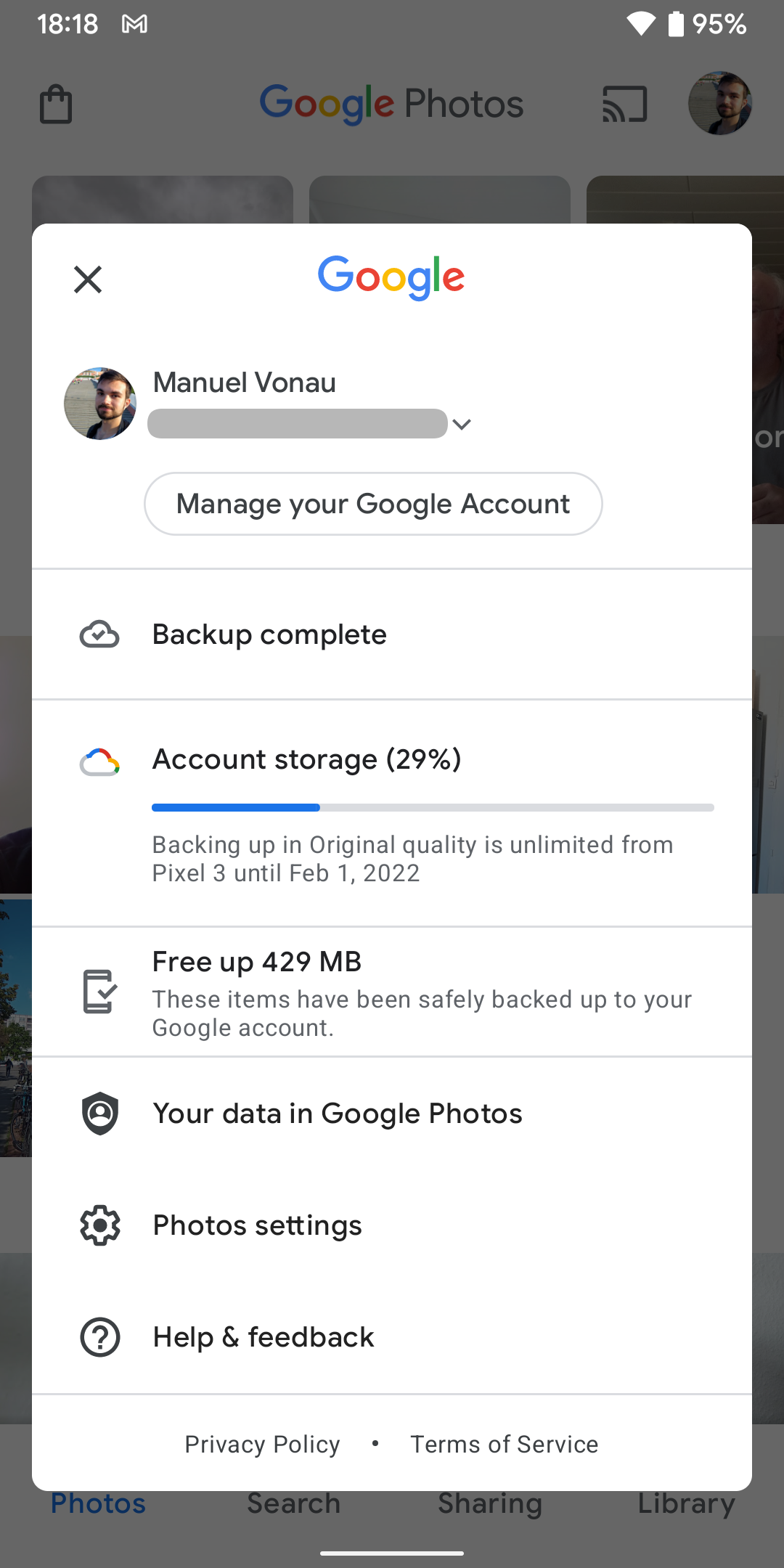Screenshot of a mobile device at 18:18. The battery is nearly full at 95%, and the Wi-Fi signal is strong. The image displays a Google pop-up interstitial featuring the multicolored Google logo at the top. Beneath the logo, it reads "Manuel Von Ahl, manage your Google account," with a button labeled "Manage your Google account." The pop-up indicates a "Backup complete" status, showing the account storage usage at 29% through a visual graph. It suggests freeing up 429 MB, noting that items have been safely backed up to the Google account. The interstitial also includes sections titled "Your data in Google Photos," "Photo settings," and "Help and feedback."